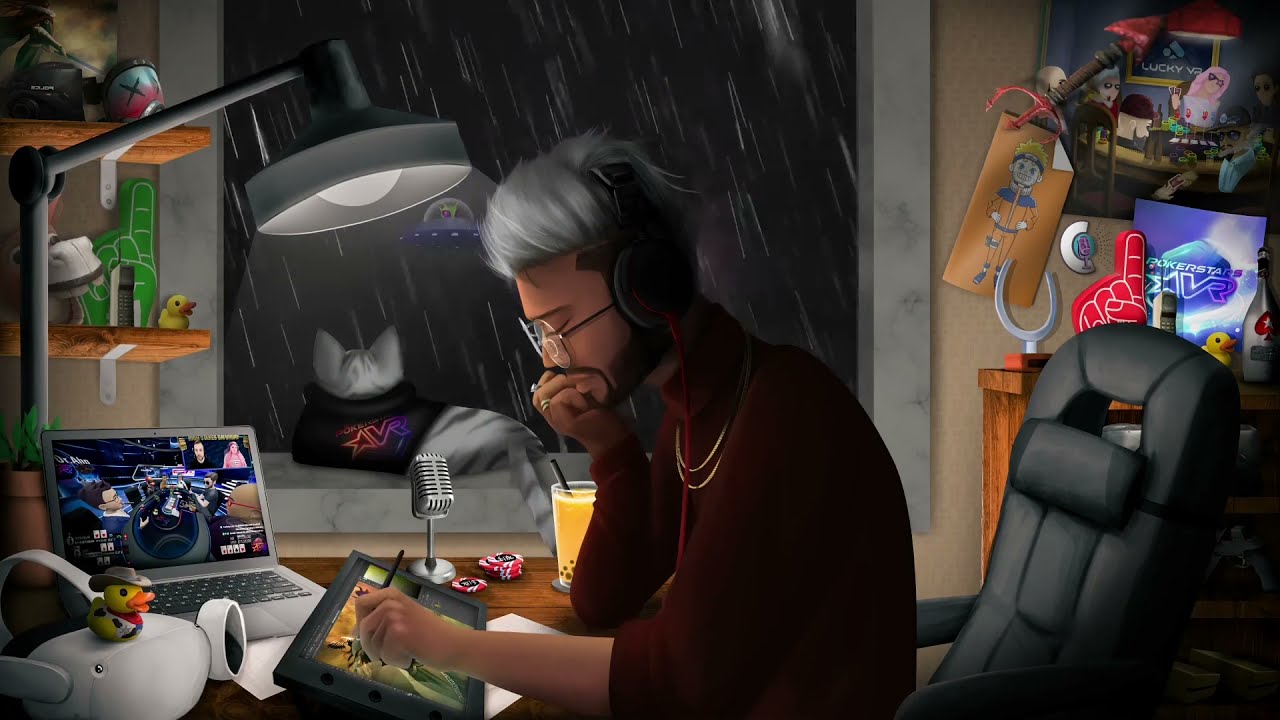The detailed computer illustration depicts a stylish man immersed in his creative work in a vibrant, eclectic studio. The man, viewed in profile from a front and center perspective, is sketching intently on an illuminated drawing tablet with a stylus in hand. He is seated in a gaming chair, dressed in a burgundy turtleneck with a gold chain, silver hair, glasses, and black headphones. To his left, a silver laptop with a game stream on its blue-tinged screen, a white VR headset adorned with a yellow rubber duck sporting a gray cowboy hat, and a boba tea with an amber hue clutter the desk. Nearby, a silver microphone and a tidy stack of red poker chips further populate the workspace. 

Behind him, a cat in a purple shirt sits on a windowsill, gazing into a stormy night sky featuring a mysterious alien saucer. Above the cat, an old-style lamp casts light, with some shelves packed with colorful trinkets, including orange and green artifacts, a foam finger, and additional rubber ducks. To his right, various posters adorn the wall. The scene, rich in color and detail, embodies a fusion of the man's creative domain and elements from a lively digital environment.